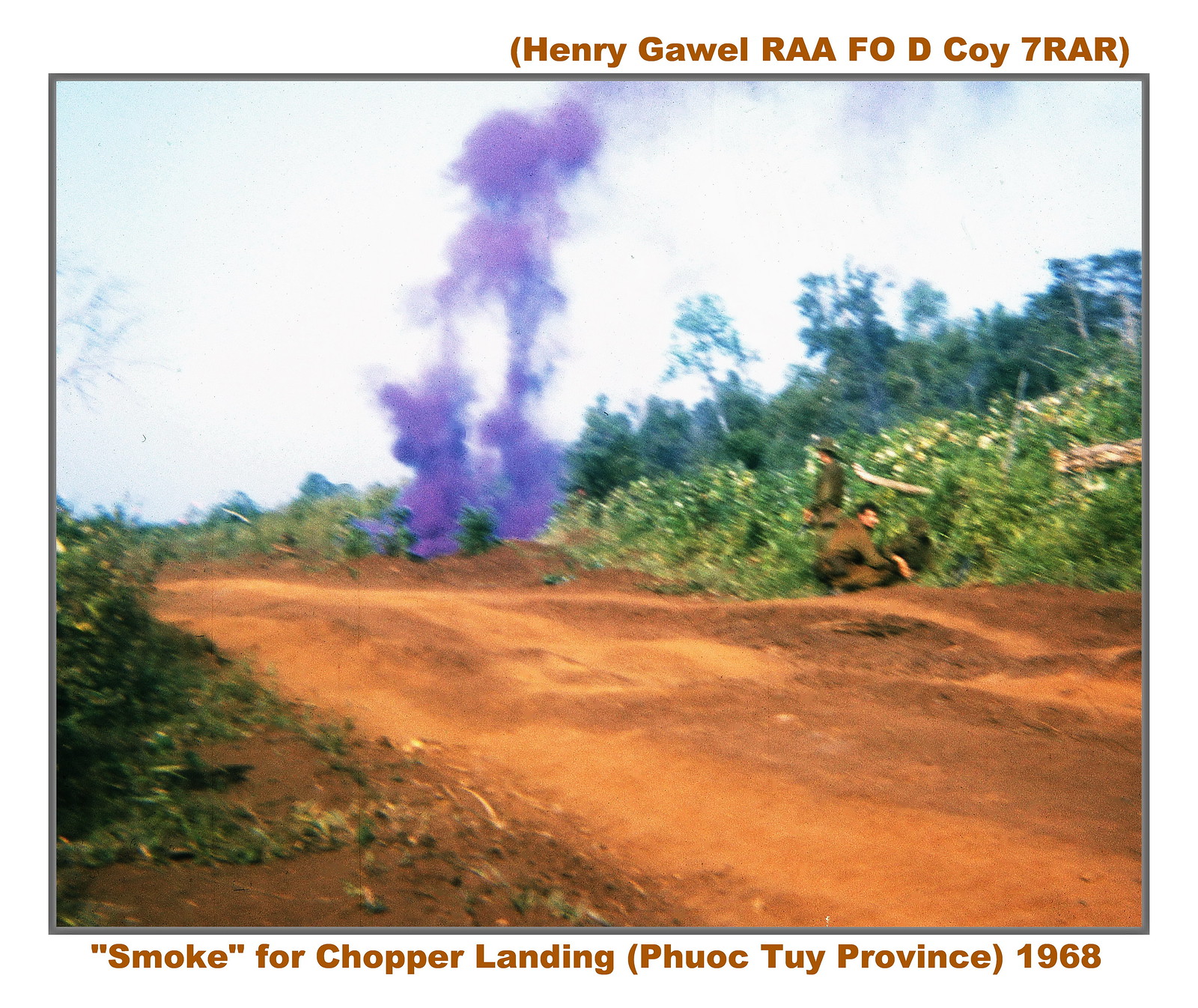The image, likely from the 1960s during the Vietnam War, shows a scene in Phuoc Tuy Province, 1968, according to the caption at the bottom. The photograph captures purplish smoke rising, presumably serving as a signal for a helicopter landing. The clear day reveals a whitish sky with a patch of blue in the distance. The vivid colors highlight a dirt road bordered by vegetation, bushes, and trees in the background. On the right side of the road, two indistinguishable men in green uniforms are visible—one standing and one kneeling amidst the foliage. Red text at the top of the image reads, "Henry Gowell RAAFO Decoy 7 RAR," though its exact meaning is unclear. The overall composition, with its vivid colors and specific details, suggests an authentic 60s-era photograph.